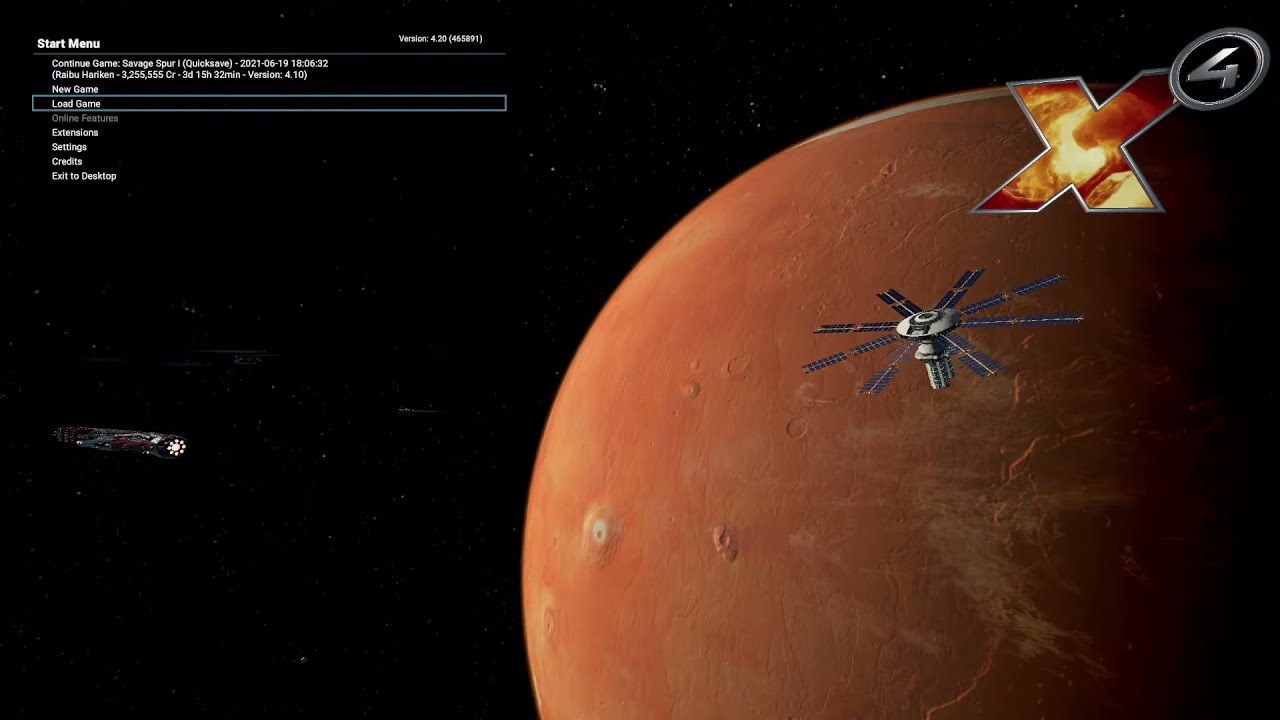The image appears to be a screenshot from the homepage of a computer game titled "X4". Dominating the right side is a large, orange planet reminiscent of Saturn or Mars, set against a predominantly black, star-speckled background suggesting outer space. In the center right foreground, a detailed spacecraft resembling a combination of a satellite and a screw with fan-like attachments is approaching the planet. To the left, another slender, tubular spacecraft with a white light at one end is either entering or exiting the scene. In the top right corner, the game title "X4" is prominently displayed, featuring a bold "X" filled with flames and a circle above the "X" containing the number 4. The top left corner includes a clearly visible start menu offering options such as "New Game," "Load Game," "Extensions," "Settings," "Credits," and "Exit to Desktop," reinforcing the idea that this is the launch screen for a space-themed video game.